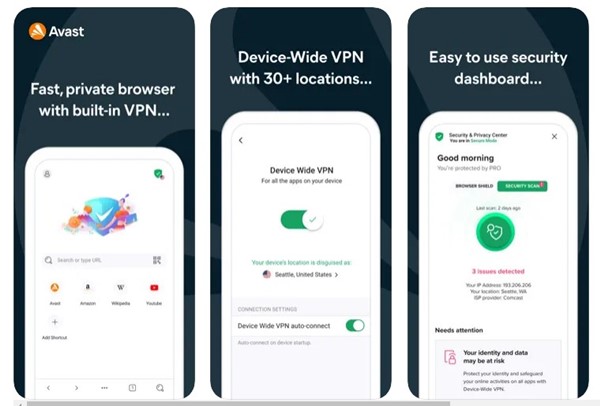**Image Caption: Comprehensive Overview of Avast's Security and Private Browsing Features**

The image is a detailed screenshot depicting three adjacent, phone-shaped interfaces, each showcasing various features of Avast's security and privacy offerings against a dark black and gray background with white vertical rectangular insets:

1. **Top Left Interface:**
   - The interface header contains "Avast" written in white, accompanied by an orange circle with a stylized "A".
   - It promotes the "Fast Private Browser with built-in VPN".
   - A visual inset presents a blue shield with a checkmark, flanked by two people seemingly holding hands.
   - Below this image, there is a search bar followed by four app icons: YouTube, Wikipedia, and two others that are indistinct.

2. **Middle Interface:**
   - At the top, it advertises "device-wide VPN with 30+ locations..."
   - The inset explains "device-wide VPN for all the apps on your device".
   - A green oval bar with a white circle showing activation status indicates that the VPN is active, displaying the text: "Your device's location is disguised as Seattle, United States" (though the words are somewhat blurry).
   - Below this, it mentions "device-wide VPN auto-connect", again accompanied by a green bar featuring a white circle.

3. **Bottom Right Interface:**
   - Heading with "easy to use security dashboard..."
   - The inset describes the "Security and Privacy Center" and greets with "Good morning, you're protected".
   - Includes a green bar and a white bar, the exact text on them is unclear, with the mention of "Browser Shield".
   - Lower down, red text indicates "Three issues detected".
   - Near the bottom, it alerts that "Your identity and data may be at risk", signaling the "needs attention" area.

This screenshot comprehensively illustrates Avast's emphasis on integrated security and privacy solutions, making it visually accessible while detailing its protective features.